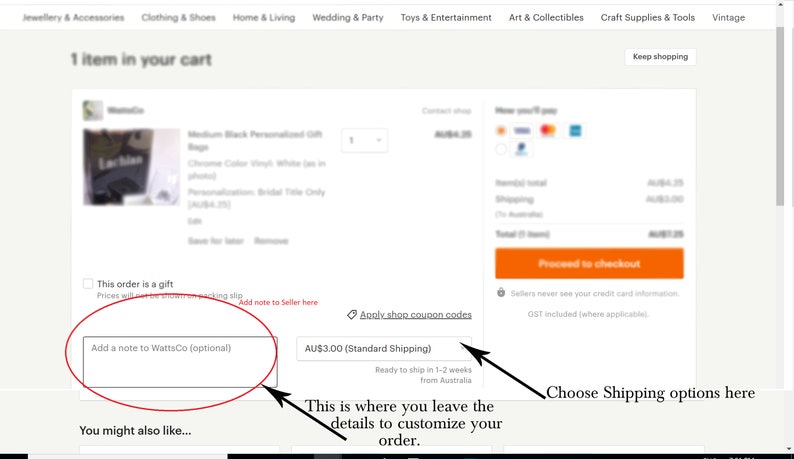In this image, we are presented with a screenshot of a shopping website's interface in an online marketplace. The top portion of the page displays several main categories, even though much of the text is blurred. From what is legible, we can identify categories such as "Jewelry and Accessories," "Clothing and Shoes," "Home and Living," "Wedding and Party," "Toys and Entertainment," "Art and Collectibles," "Craft Supplies and Tools," and "Vintage." Each category is clickable, allowing users to explore more specific options within each section.

The middle portion of the page remains blurred, obscuring some of the details. However, towards the bottom of the page, clarity improves. We see an option labeled, "This order is a gift," where users can check a box to indicate their purchase is a gift.

In the lower regions of the page, a black arrow points to a section labeled "Choose Shipping Options here," guiding the user to select their preferred shipping method. Another arrow highlights a field where users can "Add a note to What's What (W-A-T-T-S Co.)," intended for leaving customization details for their order.

In the bottom left-hand corner, there's a section titled "You Might Also Like…," presumably showcasing recommended products related to the user's interests or current shopping selections.